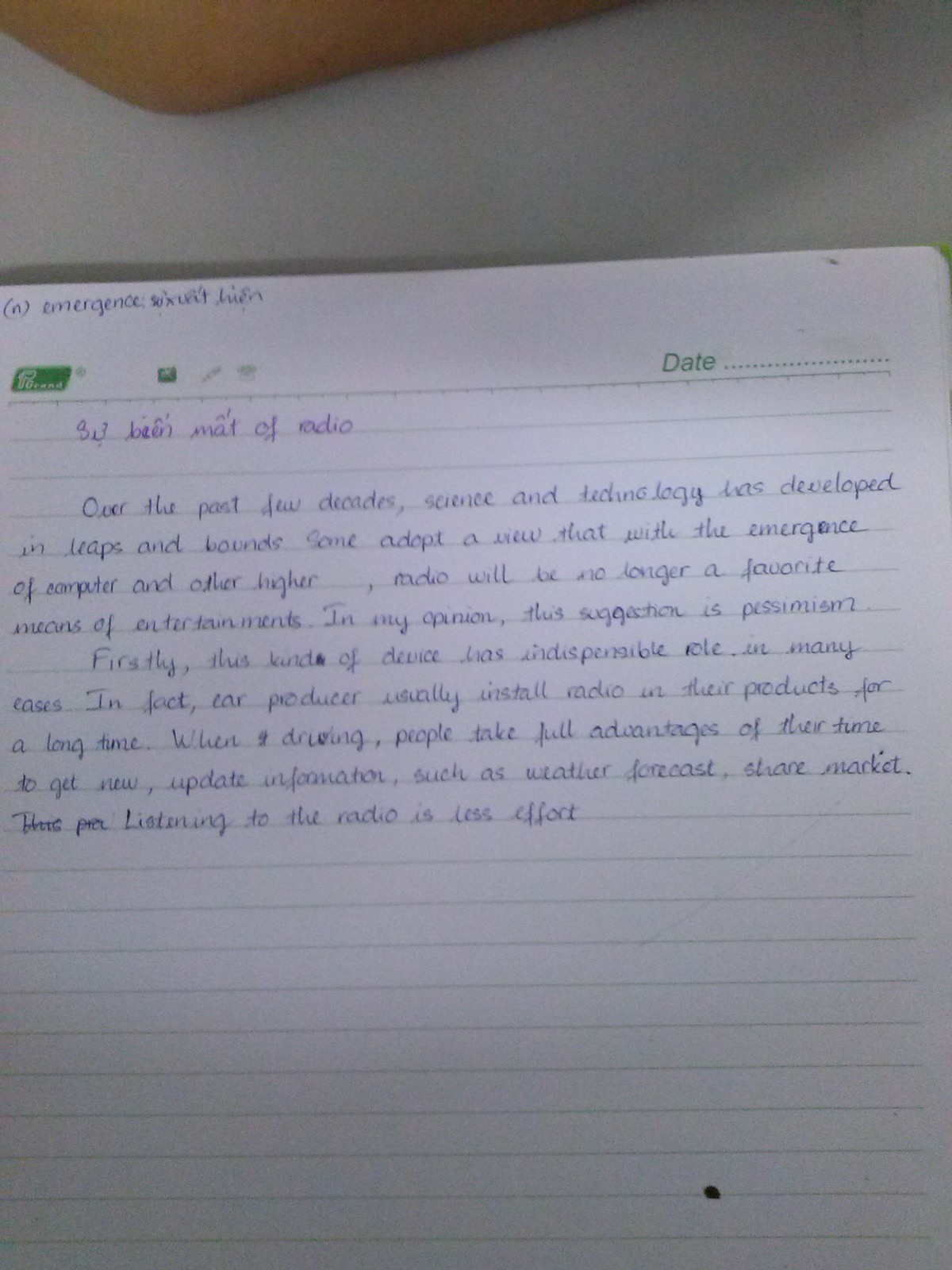A photo of a white journal page filled with blue handwriting and faint green lines. The page, undated but with a pre-printed green date section in the upper right corner, captures a handwritten entry in English. The text discusses the rapid development of science and technology over recent decades, expressing a counter-opinion to the belief that radios will become obsolete with the rise of computers and advanced technologies. The writer argues that radios have indispensable roles, especially in cars where drivers use them for updates on weather, markets, and more with minimal effort. The text is somewhat hard to decipher, with occasional missing or scratched-out words. The top of the page features some non-English writing in blue ink, and there's a small dark brown speck in the bottom right corner.